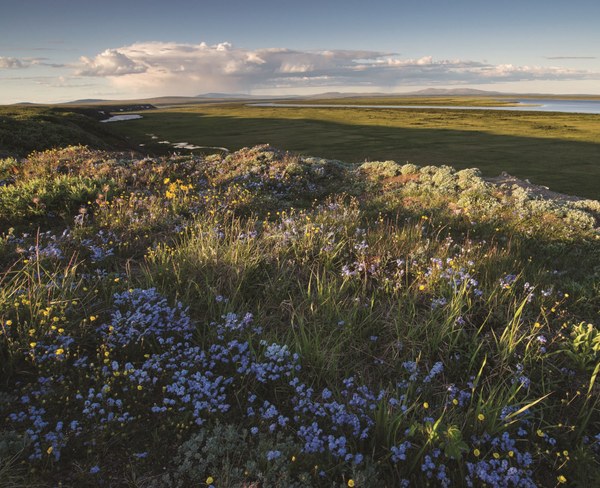This daytime landscape photo captures a vibrant meadow in intricate detail. The foreground is dotted with an array of tiny purple and yellow flowers interspersed among lush, lively green grass. As the eye travels forward, the terrain descends gently into a valley. Further back, this meadow extends into an open field of pure green grass, partially cloaked in a shadow suggesting either late afternoon or early evening light. The middle ground features a water body, likely a river or possibly a lake, faintly visible before leading the eye to the horizon. Beyond the water, distant mountains loom faintly against a sky filled with an assortment of clouds, ranging from wispy white to darker gray hues, some suggesting rain. The light creates interesting contrasts, illuminating certain plant life while casting others into shade, adding depth to the serene landscape.